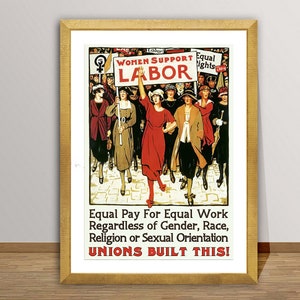In this picture, we see a detailed and vibrant framed painting, leaning against a white wall on a hardwood floor with a hardwood baseboard. The frame is light brown, and the painting itself is bordered with white. The scene within the painting depicts a spirited women's support labor rally, where numerous women are assembled, each holding various signs. The central figure of the painting is a woman dressed in a striking red gown and matching red shoes, with a hat on her head, and one hand raised. The signs these women hold are bold and prominently feature messages such as "Women Support Labor" in red, capital letters, "Equal Rights," and "Equal Pay for Equal Work regardless of gender, race, religion, or sexual orientation." Adding to the call for equality, a red sign with a fist and gender symbol is on the top left. The diversity and solidarity of the women are highlighted by their varied attire, ranging in colors from red to brown to yellow to maroon. Underneath the bustling rally scene, the painting features the phrase, "Unions Built This!" in emphatic red font. This artwork captures the essence of a powerful movement advocating for labor rights and equality.